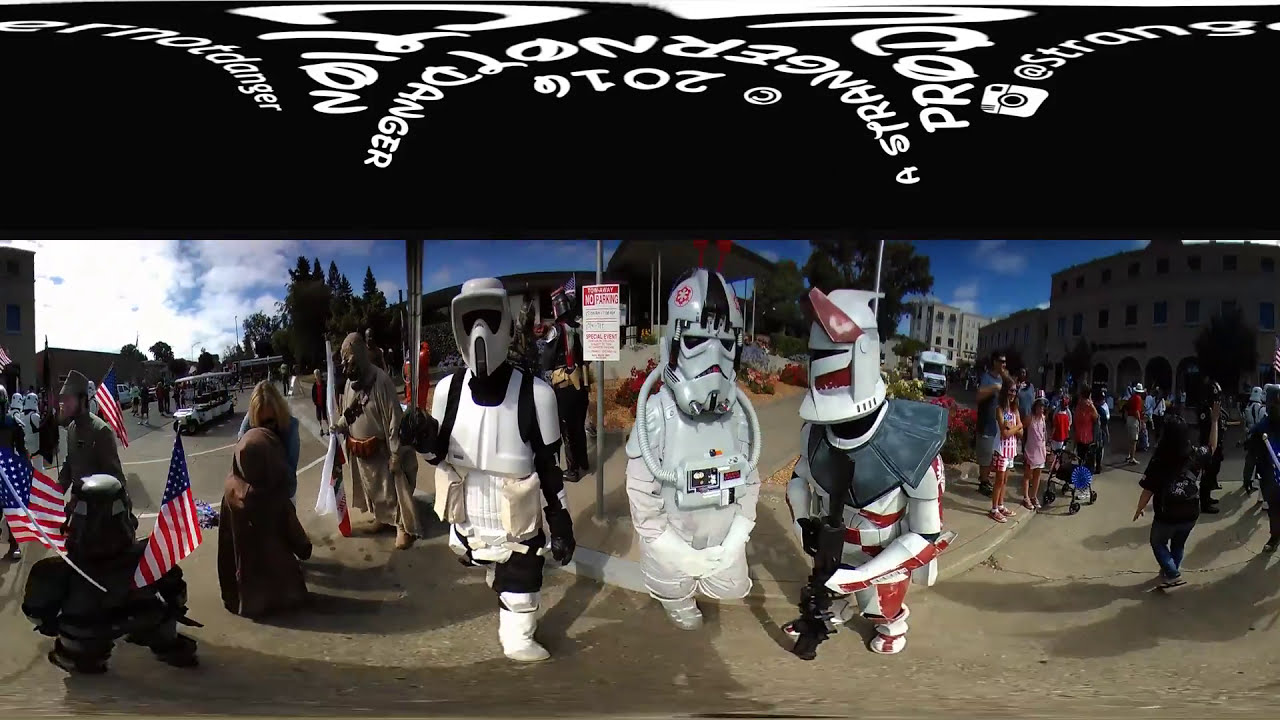The photograph captures an outdoor scene that resembles a festival or Star Wars convention. Dominating the center, three individuals dressed as stormtroopers stand on a dirt ground in front of a 'No Parking' sign; each costume is slightly different, with the rightmost one featuring black and red elements. To their left, another person donning a Star Wars robe can be seen, while several others, some in costumes and others not, are scattered around the scene. The background features a large building with numerous windows on the right, while the left side showcases a clear blue sky with clouds. American flags are visible, being held by people along the roadside where golf carts or small trucks are driving. The atmosphere hints at a celebratory event, possibly linked to the 4th of July, with additional bystanders observing the scene.